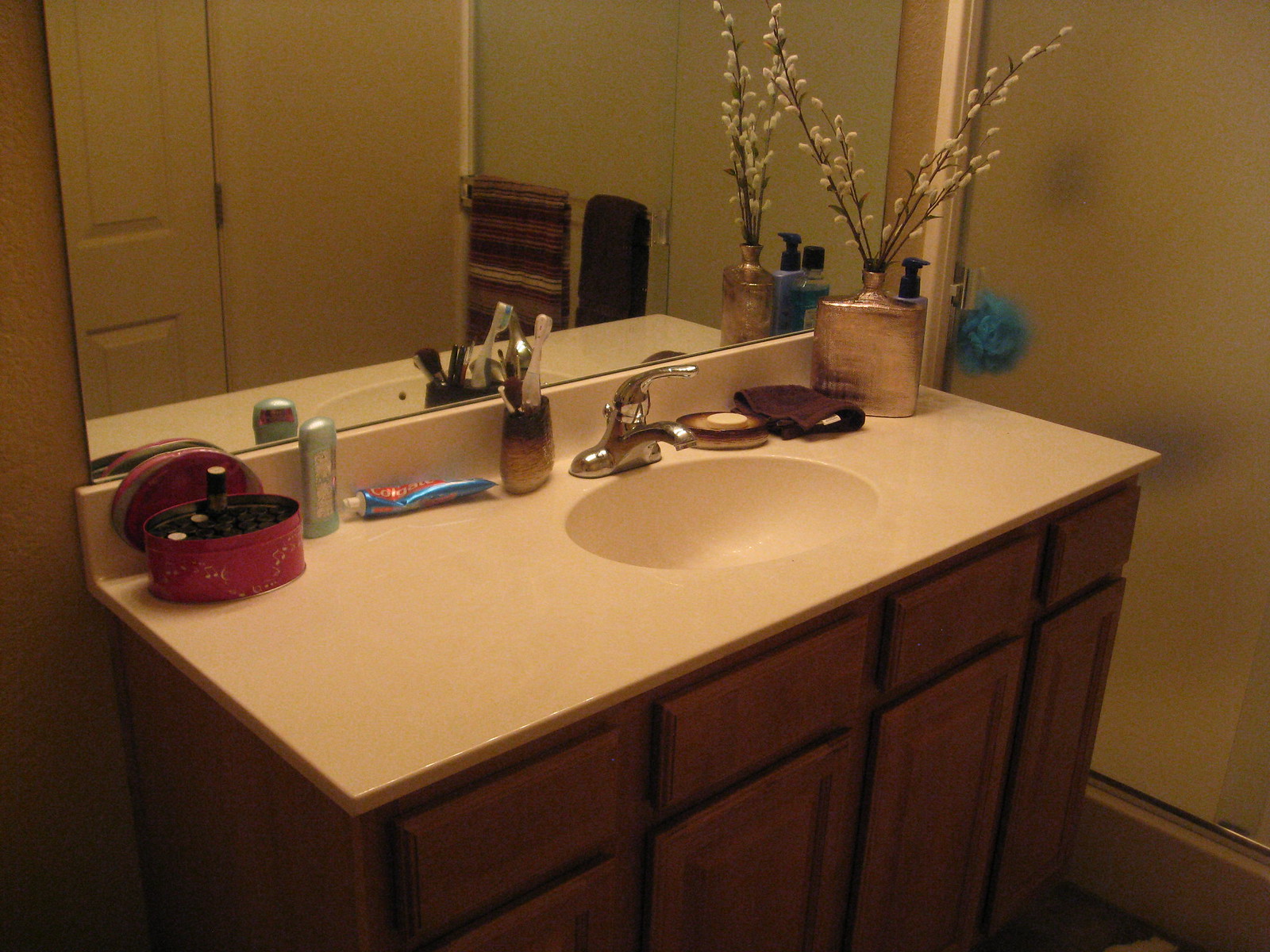The photograph captures a small, elegantly arranged bathroom sink. The sink, crafted from a white marble-like porcelain, rests atop a beautifully stained wooden cabinet. The wooden base features a combination of four drawers and four cabinets, providing ample storage space beneath the sink.

On the countertop sits an assortment of personal items. A vibrant red, oval-shaped makeup box stands out prominently. Next to it, a light blue, almost fluorescent deodorant adds a touch of color. Nearby, a tube of blue and red toothpaste is placed next to a brown to beige toothbrush holder, slightly oval in shape and wooden in appearance, containing various toothbrushes.

The sink's handles are a sleek, silvery round design, contributing to the contemporary feel of the space. A matching soap dish, brown and cream colored like the toothbrush holder, is thoughtfully placed beside the sink. Adjacent to the soap dish, a brown hand towel complements the overall color scheme, tying the different elements together.

Adding a touch of natural beauty, a small bronze vase containing delicate white Baby's Breath flowers is positioned nearby. The flowers, on dark or black stems, provide a subtle contrast to the otherwise earthy tones of the decor. 

In the background, the edge of a shower can be faintly seen, with a loofah hanging on the wall and a clear shower door indicating the clean, modern design of the bathroom. The cohesive palette of light brown, dark brown, cream, and hints of bronze creates a warm, inviting atmosphere.